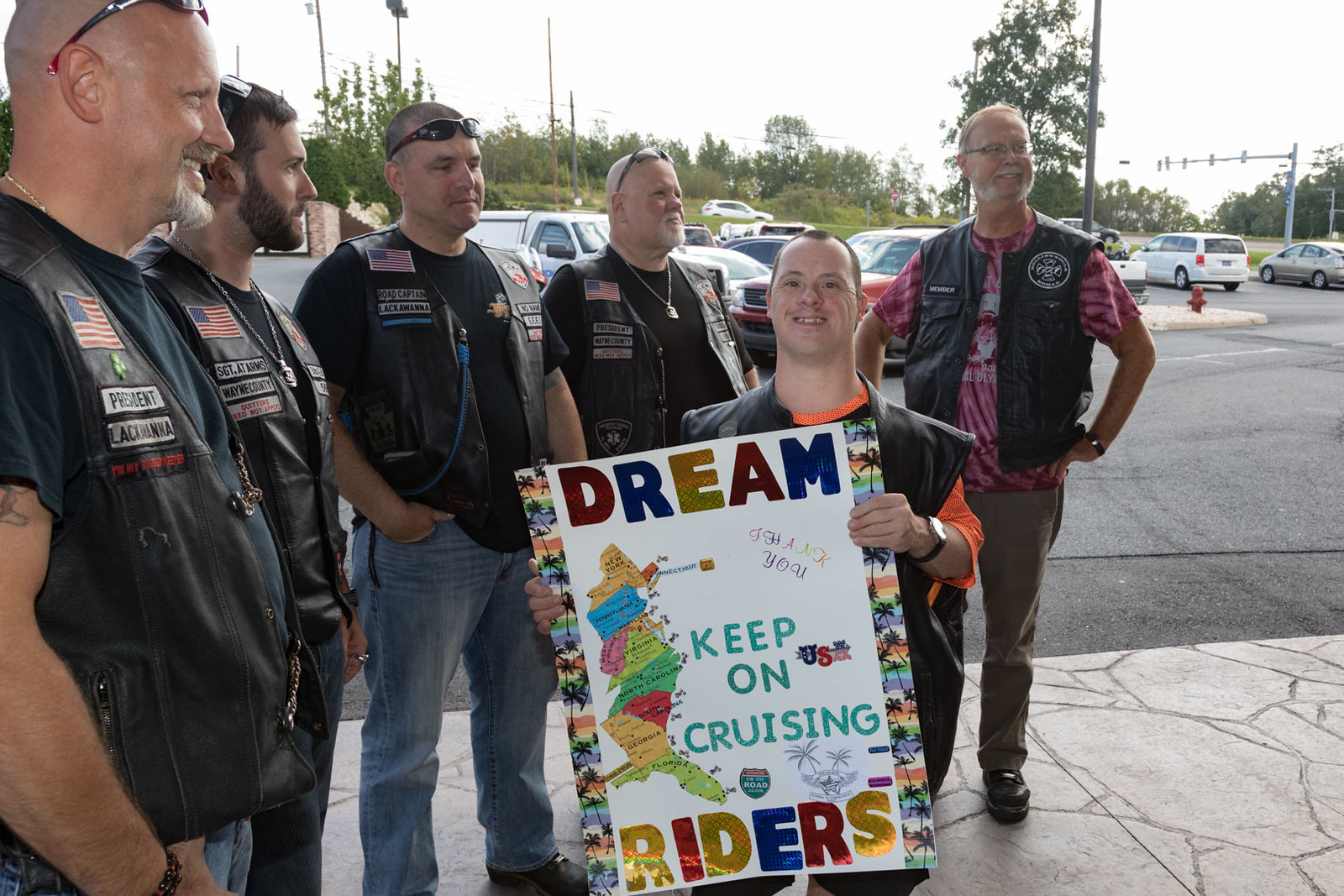In this image, six people are standing on a sidewalk next to a parking lot, with a road and a streetlight visible in the background. Five of the individuals are wearing black vests adorned with the United States flag on the left side and a badge on the right side, with one of them bearing the title “President.” They are dressed in black shirts and denim pants, except the person on the far right who is wearing a stylized pink shirt and dark brown pants. All but one are wearing sunglasses. 

In the foreground, at the center of the group, is a man with Down Syndrome, wearing a black vest over an orange shirt. He is holding a poster that reads "Dream Keep on Cruising Riders" in large, colorful, capital letters that are shiny in hues of red, blue, and gold. The poster also features a multicolored map on the left side, displaying various states in colors like red, green, yellow, orange, and pink. The poster’s border consists of a pine tree silhouette with red, green, and blue colors on the left and right sides. Everyone appears pleased, suggesting a moment of shared accomplishment and camaraderie, possibly part of a make-a-wish event.